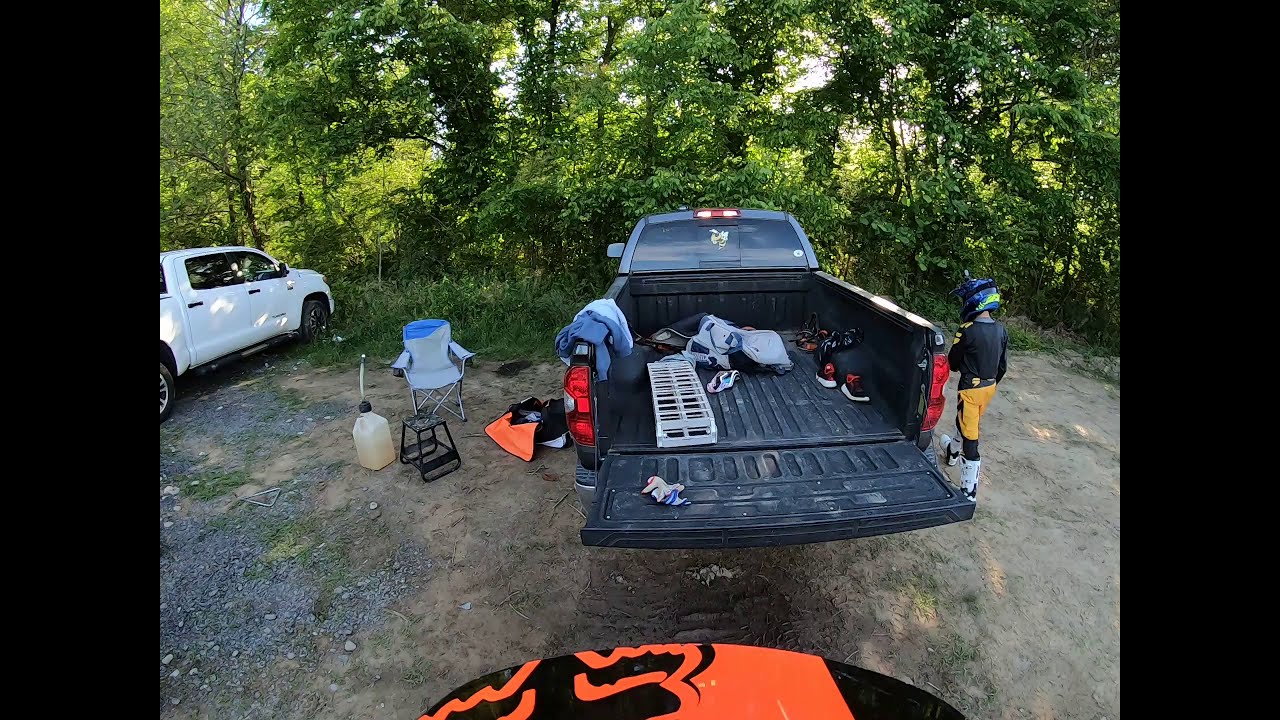The image shows a serene yet slightly cluttered forested area with dense green trees and sunlight filtering through. Prominently positioned in the middle is a gray pickup truck with its back gate open, showcasing a black-lined truck bed containing black shoes and various clothing items. To the left side of the image, another white pickup truck is partially visible. 

On the ground between the two trucks lie several items: an open lawn chair, a black stool, and a large plastic jug, possibly for gasoline, with a tube sticking out. An open bag with an orange interior is also present. A young individual, likely a teenager, stands to the right of the gray truck, wearing a blue and yellow helmet, a black long-sleeve shirt, yellow pants, and white shin guards or tall boots. The gravelly gray ground beneath them emphasizes the outdoor setting, complemented by the surrounding tall grass and heavy foliage in the background. The entire scene is framed by large black bars, typical of a photo taken on a cell phone.